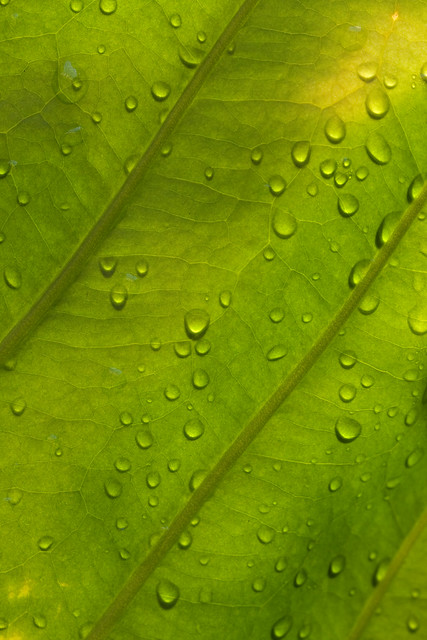This close-up photograph showcases a vibrant green leaf, bathed in early morning sunlight, adorned with around fifty sparkling water droplets. The leaf exhibits varying shades of green, from lime to medium, with a detailed network of veins prominently visible. These veins, two of which are darker olive green and run vertically, structurally divide the leaf into three distinct sections. Each section is filled with intricate, lighter-colored veins that resemble the spreading roots of a tree. The water droplets, displaying a range of shapes from circular to pear-shaped, hint at their gradual downward movement, casting gentle shadows that enhance the leaf's texture and the overall impression of freshness and vitality.